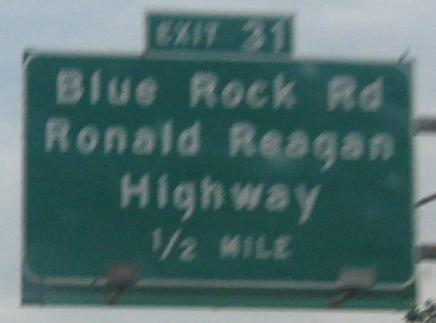This is a daytime photograph of a freeway sign, tightly cropped to show just the sign. The background of the sign is dark green with a white border. The main panel of the sign features large white text that reads, "Blue Rock Road Ronald Reagan Highway 1/2 Mile." Below this, there are several lamp poles extending downwards, although they are not illuminated. Above the main panel is a smaller, rectangular sign with a matching dark green background and white border, displaying the text "Exit 31." To the right of the sign, metal poles are visible, which support the sign structure. The sky in the background appears overcast, with a mix of light blue tones and wispy white clouds. The image quality is grainy and blurry, indicating it may be of low resolution. There is no other subject matter or elements present in the image.